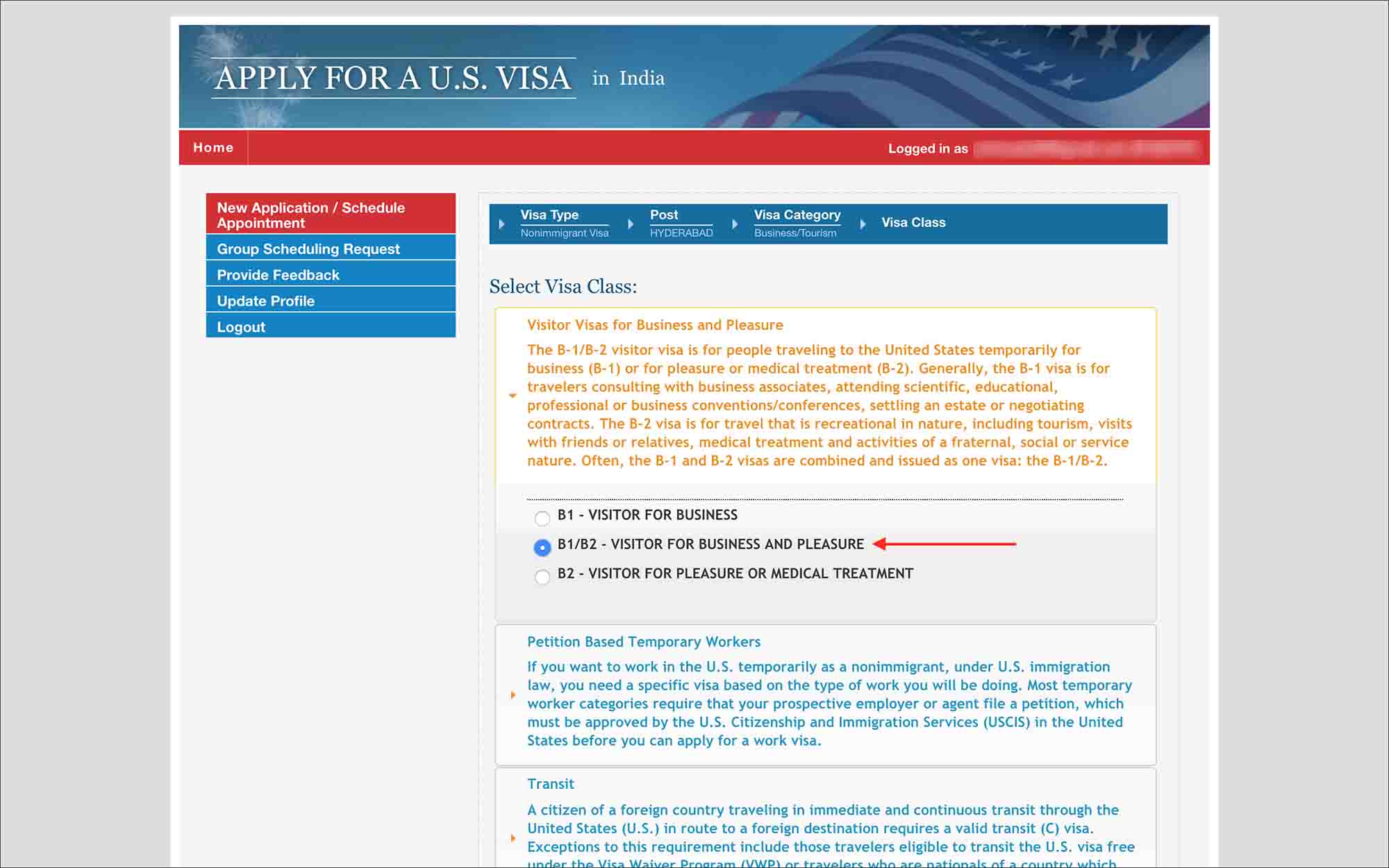Under the heading "Websites," the page features a prominent blue bar at the top, emblazoned with the text "Apply for a U.S. Visa in India." A piece of the American flag, depicted as floating amidst clouds, is positioned above this blue bar. A red line underscores this section. Below, in white letters, it reads "Home" and "Logged in as," though the login name is blurred for privacy.

In the next section, "New Application" and "Schedule Appointment" are written in bold red text. The options "Group Scheduling Request," "Provide Feedback," "Update Profile," and "Logout" follow, presented in teal text with white letters. Adjacent to these options, a series of dropdown menus and labels are located. The labels include "Visa Type," listed as "Non-Resident Non-Immigrant Visa," and "Post," specified as "Hyderabad." Additionally, "Visa Category" is recorded as "Business/Tourism."

Directly below is a dropdown menu under "Select Visa Class," where orangey-red text indicates various options. The description elaborates that the B-1/B-2 Visitor Visa is meant for individuals traveling to the United States for specific temporary purposes. The B-1 visa is primarily for travelers visiting for business-related activities, such as consulting with business associates, attending scientific, educational, professional, or business conventions or conferences, settling an estate, or negotiating contracts. For those traveling for pleasure or medical treatment, the B-2 visa is applicable.